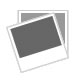This is a detailed color photograph depicting a charming wall sconce in a minimalistic setting. Mounted on the pristine white wall is a rectangular wooden platform with a smaller triangular support piece below it. The wood, possibly vintage in appearance, casts a noticeable grayish shadow against the wall, adding depth to the image. Atop the wooden shelf sit two light tan ceramic cat figurines, exuding a nostalgic charm. The first cat lies down with its tail curled around itself, while the second cat, with its tail characteristically straight up, sits next to it, paws playfully placed on the lying cat's ears. The cats, facing slightly different directions, have dark eyes which add a touch of detail. The photograph, likely taken with a flash given the clear reflections on the wall and the shelving, captures the peaceful simplicity of this vintage display, suggesting an intimate domestic setting devoid of additional text or embellishments.